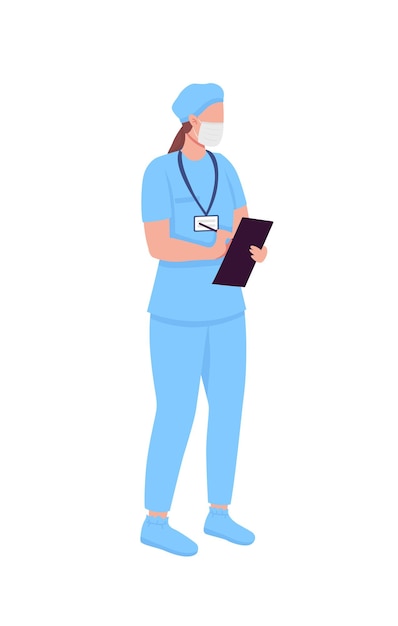The illustration depicts a female nurse with brown hair pulled back into a ponytail, wearing a blue scrub cap and a white surgical mask that obscures her facial features. She is dressed in blue scrubs with a short-sleeved top, long pants, and blue booties with darker soles. Around her neck hangs a black lanyard with a white identification badge. In her right hand, she holds a black pen, and in her left hand, a rectangular black tablet on which she is writing. The nurse's skin is pale with a fairish pink hue, and the background of the image is completely white. The illustration is simple, focusing on the figure of the nurse without detailed facial features.